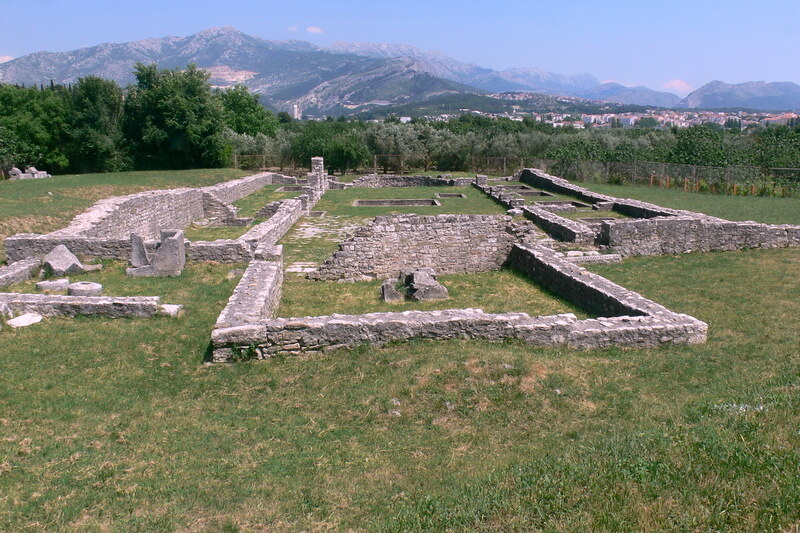The image showcases an expansive grass field, home to the remnants of an ancient stone foundation, likely the ruins of a historical or archaeological site. The remnants include parts that jut out symmetrically, hinting at a once grand stone complex now reduced to low walls and old steps, possibly dating back thousands of years. These ruins are surrounded by a serene landscape, with multiple trees lining the horizon and a city or town visible, especially towards the right side of the field. Beyond the immediate environment, a majestic mountain range stretches across the background, featuring a palette of green and brown with rocky gray peaks, under a vividly clear blue daytime sky. The distant mountains seamlessly blend into the scenery, adding depth and emphasizing the natural beauty that frames this historical site.